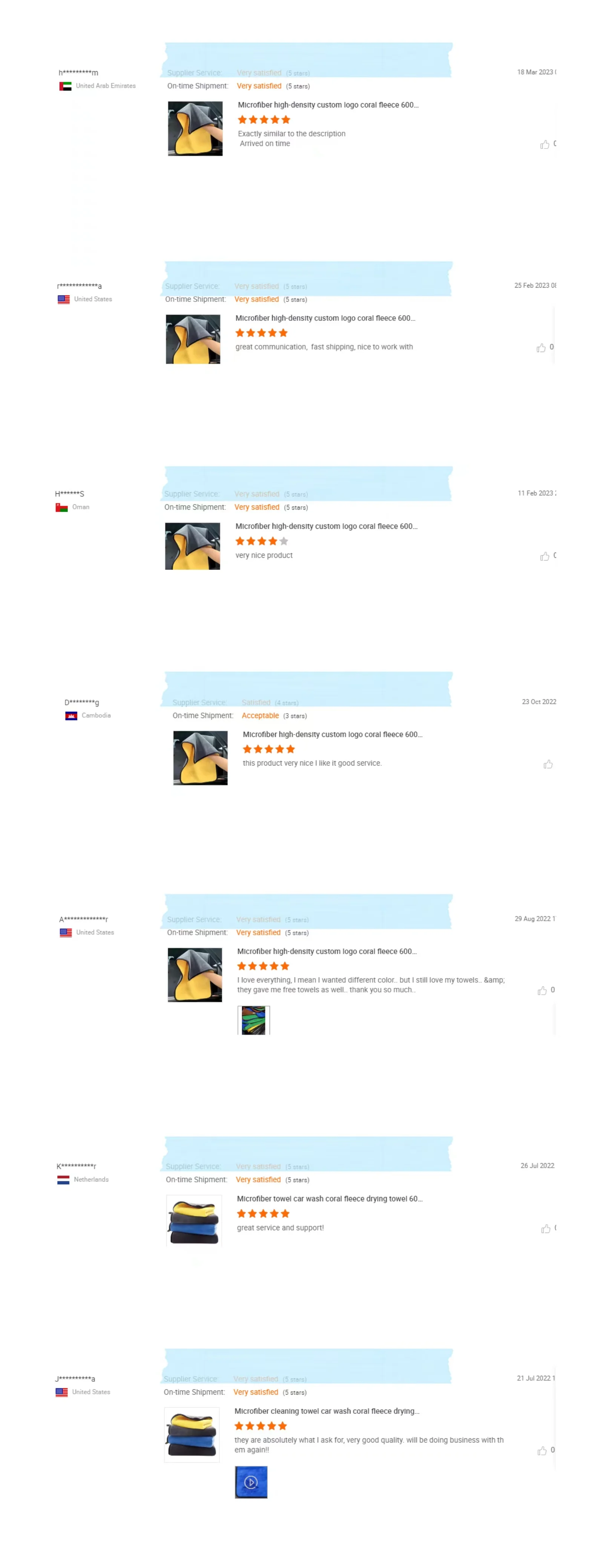The image features a white background with seven small blue boxes, each accompanied by a picture and detailed product information in very fine print. To the left of each blue box is a small icon, followed by a product image and star ratings. The first blue box shows a product with a five-star rating. The second box displays the same product but with a four-star rating. The third and fourth boxes also showcase products with five-star ratings. Beneath the fourth blue box is a tiny additional box. The fifth and sixth blue boxes feature images of towels, both rated with five stars. Beneath the sixth box, there’s another small blue box. On the far right side, extremely small text appears, likely indicating a quantity selection box for ordering the products.